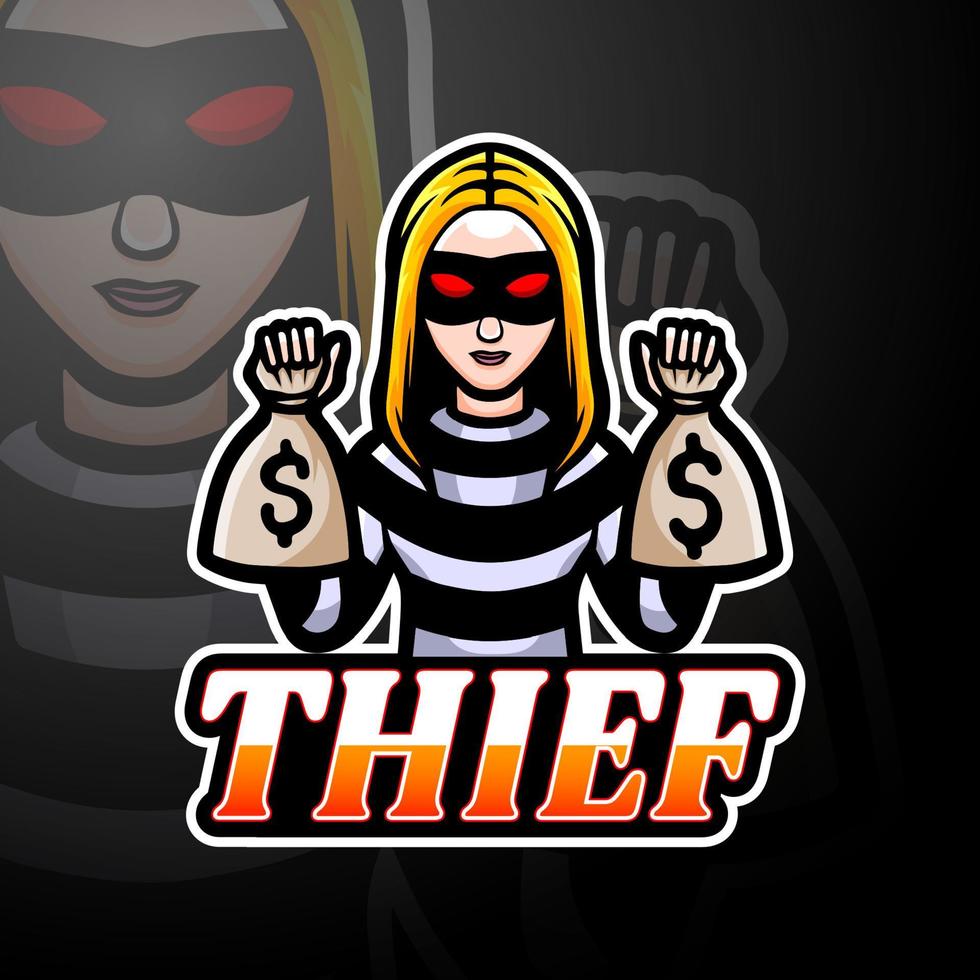This detailed illustration features a central cartoon graphic of a female thief against a black background. The main character, positioned at the center, is a blonde woman with long hair parted in the middle, wearing a black face mask that masks her eyes, which are notably red and styled like cat eyes. Clad in a black and white striped long-sleeve shirt, she holds a beige money bag in each hand, each distinctly marked with a dollar sign. Her facial expression includes a subtle, knowing half-smile, and her gaze is directed towards the viewer.

Beneath this character, in bold italicized capital letters, is the word "THIEF." The typography is distinctive, with the tops of the letters in white and the bottoms in orange, all surrounded by a white frame outline that gives the text a bold, graphic look. This frame continues around the edge of the entire image, further defining the illustration.

In the image's background is a faded, larger shadow of the same woman, subtly positioned to the left, adding depth and emphasizing the central figure. The contrast of the dark background and the vivid details of the character strongly highlight the thief as the focal point of the illustration. The entire composition, from the spotlit thief to the bold typography, is designed with a striking, sticker-like, graphic quality, making it both eye-catching and memorable.